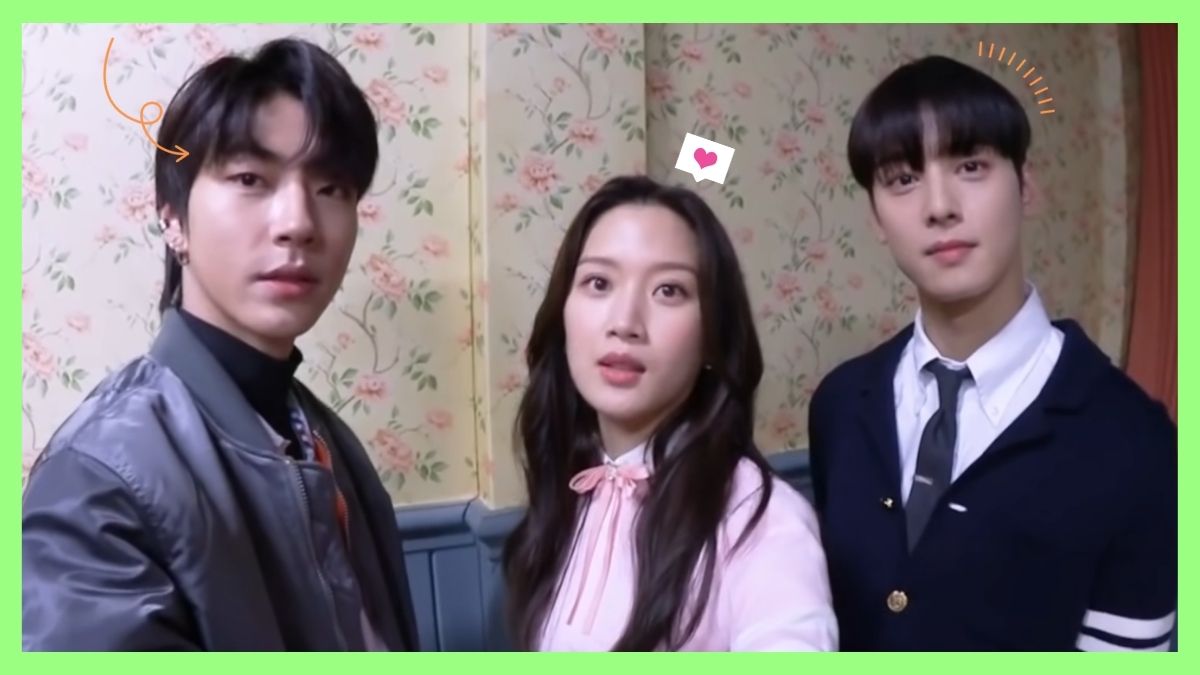The image features three people of Asian descent standing in a hallway adorned with tan and peach-colored paper wallpaper decorated with small pink flowers. On the left is a Korean man with short hair and a black leather vest; an orange, curly arrow points to his face. In the middle stands a woman with long black hair cascading past her chest, wearing a pink blouse with a high collar and a small bow, with a speech bubble containing a heart hovering above her head. On the right is another Korean man with a short bob haircut. He is dressed in a white button-up shirt, a black tie, and a black coat, with orange lines around his head indicating excitement. They appear to be posing, possibly as part of a K-pop group.